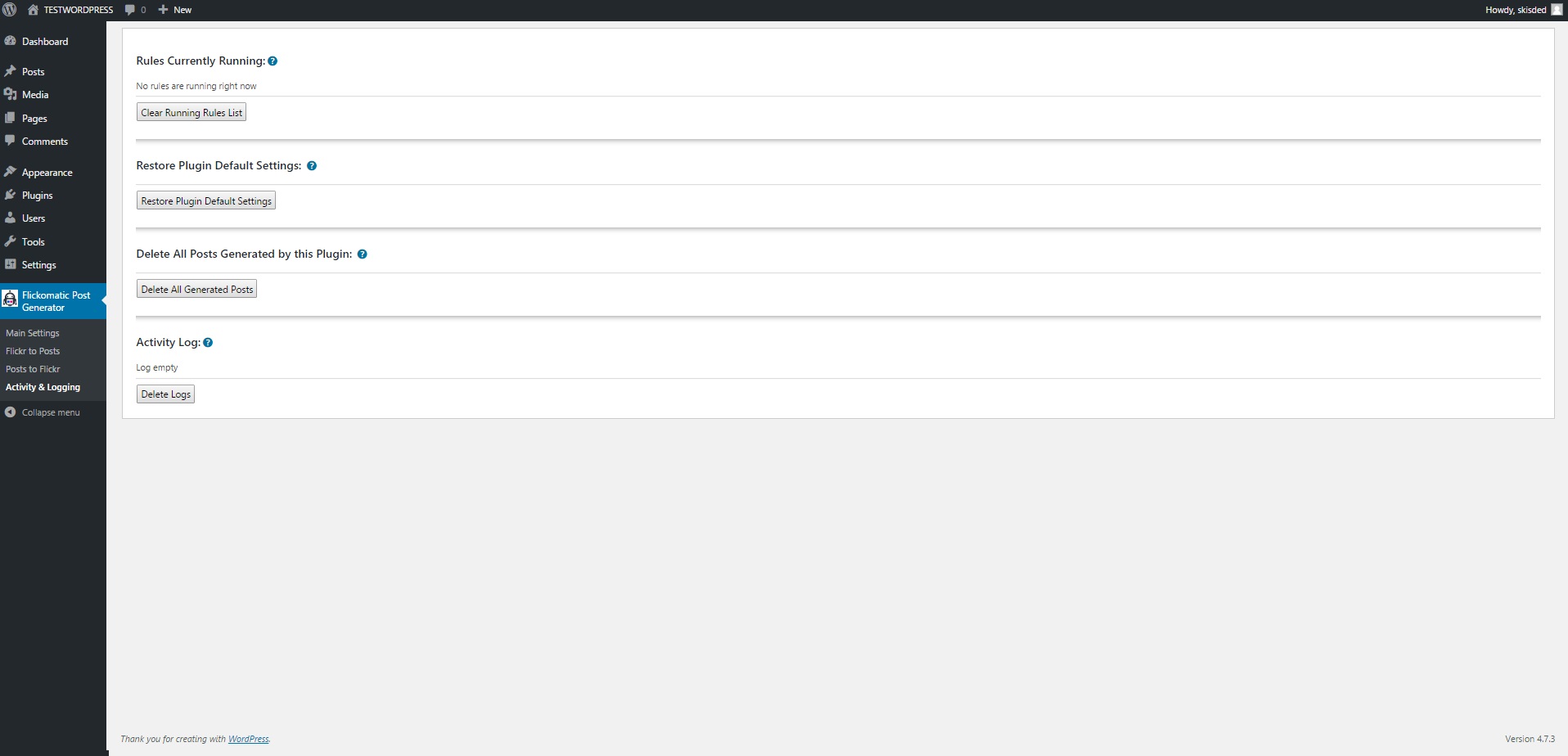The horizontally rectangular image is a screenshot of a WordPress admin dashboard, providing an overview of plugin management. The top of the image features a thin horizontal black banner, characteristic of the WordPress interface. To the left, a narrow vertical sidebar with a black background lists various menu options such as Posts, Comments, Appearance, Plugins, and Users.

One of these options is highlighted in blue, indicating it is currently active. The main content area to the right details the selected plugin’s settings and controls. Displayed options include:

- **Rules Currently Running:** Displays ongoing rules with a button labeled "Clear Running Rules List."
- **Restore Plugin Default Settings:** A button with the same label provides the option to revert settings back to their defaults.
- **Delete All Posts Generated by the Plugin:** Accompanied by a similarly labeled button for easy content removal.
- **Activity Log:** Indicates the log status with "Log Empty" and includes a "Delete Logs" button for clearing the activity records.

This detailed layout and functionality are indicative of a typical WordPress plugin management interface.